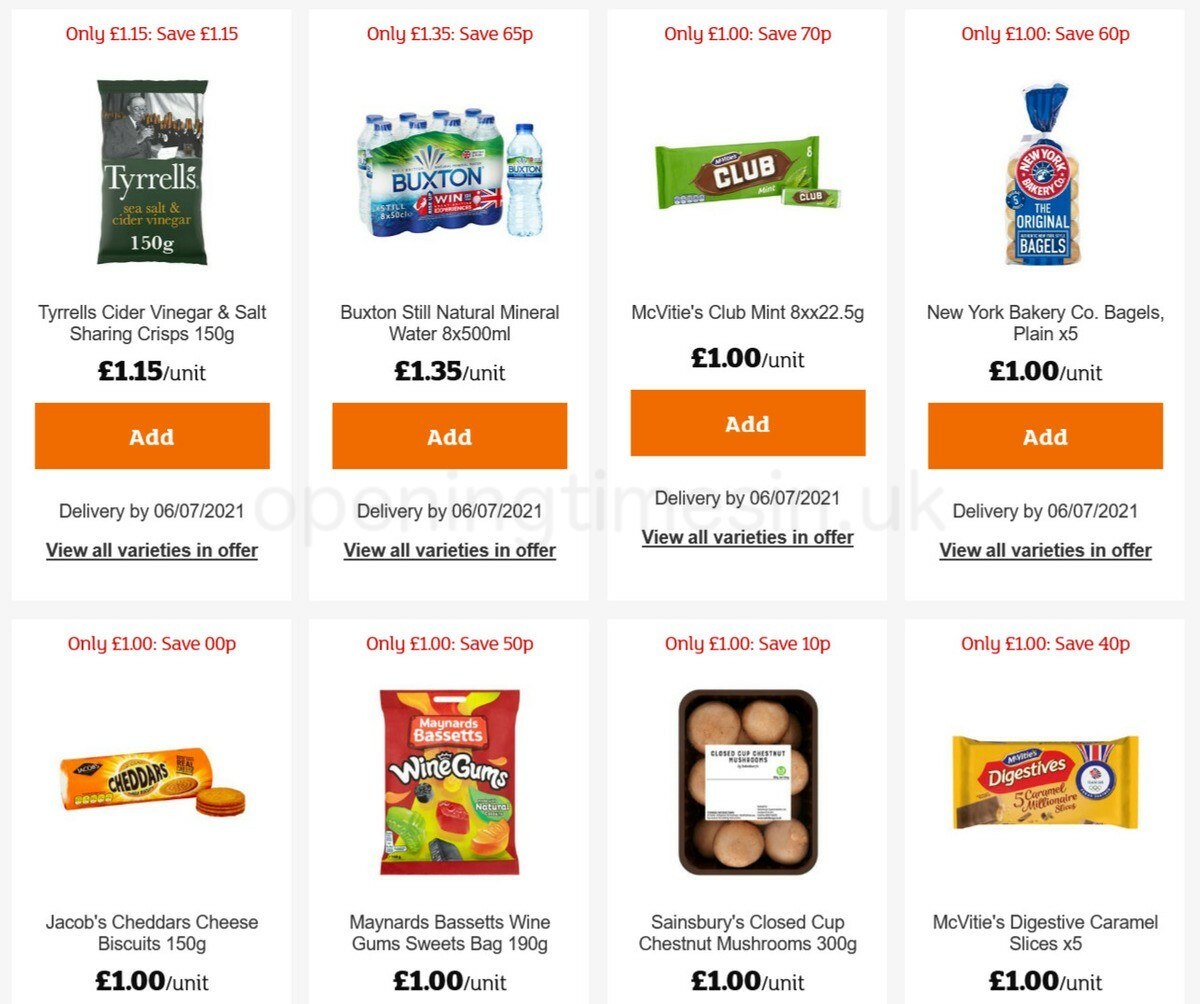This vertical image is a screenshot of an online shopping cart from a computer or smart device, showcasing various products available for purchase. The background of the image is predominantly white, accented with a light gray outline that segments each product, except at the bottom where the white blends seamlessly into the screen.

At the top of the image, there's a header showing the text "Only 1.15 pounds, Save 1.15," accompanied by an icon of Tyrell Sea Salt and Cider Vinegar Chips. Below the icon, a detailed description reads: "Tyrell Cider Vinegar and Salt, Sharing Crisps, 150 grams," and the price in bold black is stated as "1.15 pounds/unit." An orange "Add" button is visibly present, indicating the option to add the item to the cart, with a noted delivery date by "6-7 of 2021." Beneath this, there's a black underline link with the text "View all varieties in offer."

The following items, each similarly outlined and detailed, include:

1. **Buxton Still Mineral Water**
2. **McVitie's Club Mint**
3. **New York Bakery Company Bagels, Plain (x5)**
4. **Jacob's Cheddar Cheese Biscuits**
5. **Maynard's Bassett's Wine Gum Sweets Bag**
6. **Sainsbury's Closed Cup Chestnut Mushrooms**
7. **McVitie's Digestive Caramel Slices (x5)**

Each product listing is formatted consistently, with an icon, description, price, and available actions, making it easy for users to browse and add items to their online shopping cart.